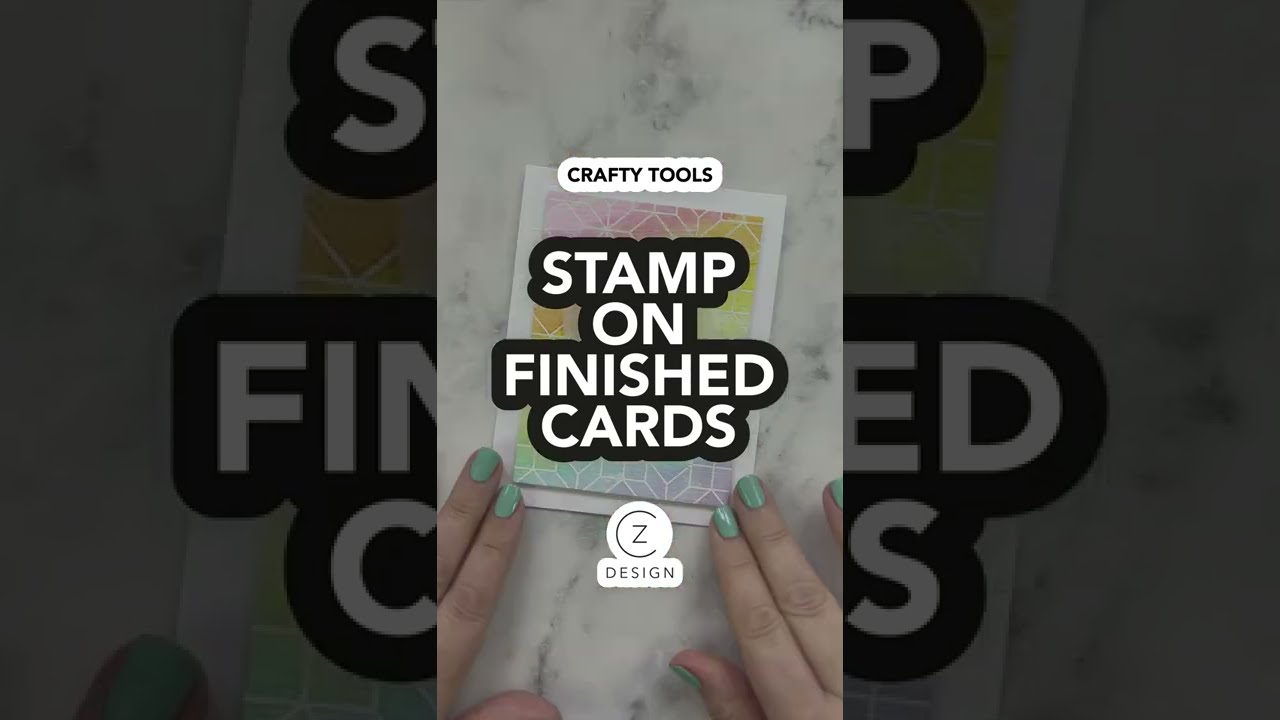The image appears to be a vertically-oriented screenshot from a how-to video. The central focus is a brightly colored greeting card with shades of pink, yellow, green, and purple, set against a white and gray stone marble tabletop. At the top of the card, there's a horizontal white oval logo with black text that reads "Crafty Tools." Just below this, in prominent white letters outlined in black, the text states "Stamp on Finished Cards." Further down, a logo displaying "CZ Design" is visible. At the bottom of the image, two hands with green fingernail polish are seen, with fingers gently touching the bottom corners of the card, suggesting careful placement or adjustment of the card. The surrounding panels of the image are darkened, directing attention to the illuminated central panel, enhancing the focus on the hands and the card.